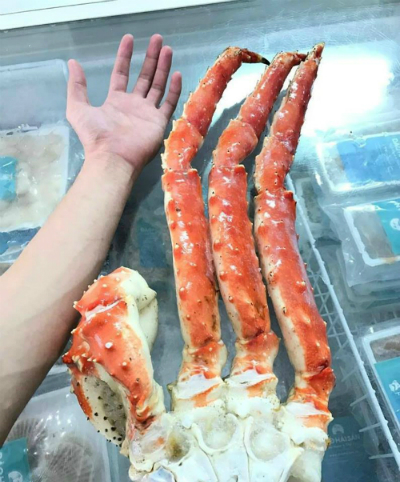This indoor photograph, likely captured in a store setting, showcases a striking display of king crab legs beside a human hand for scale. Centered in the image is a cluster of red and white king crab legs, with the crab's body or knuckle, prominently white, at the base. From this knuckle, three long, prickly red legs extend vertically, each tipped with a bent claw to the left of the knuckle. A human hand, palm up and stretched out, lies adjacent to the crab legs, highlighting their impressive length, which nearly matches the distance from hand to elbow on the human arm. The scene rests atop a glass surface, possibly a freezer, revealing various frozen products beneath, such as packaged seafood items like oysters or mussels. The background features cage-like white containers holding these packages, adding to the commercial ambiance of the setting. The dominant colors in the photo are the orange-red of the crab legs, the white of the crab's body and containers, and the blue and green hues of the packaging and surface.